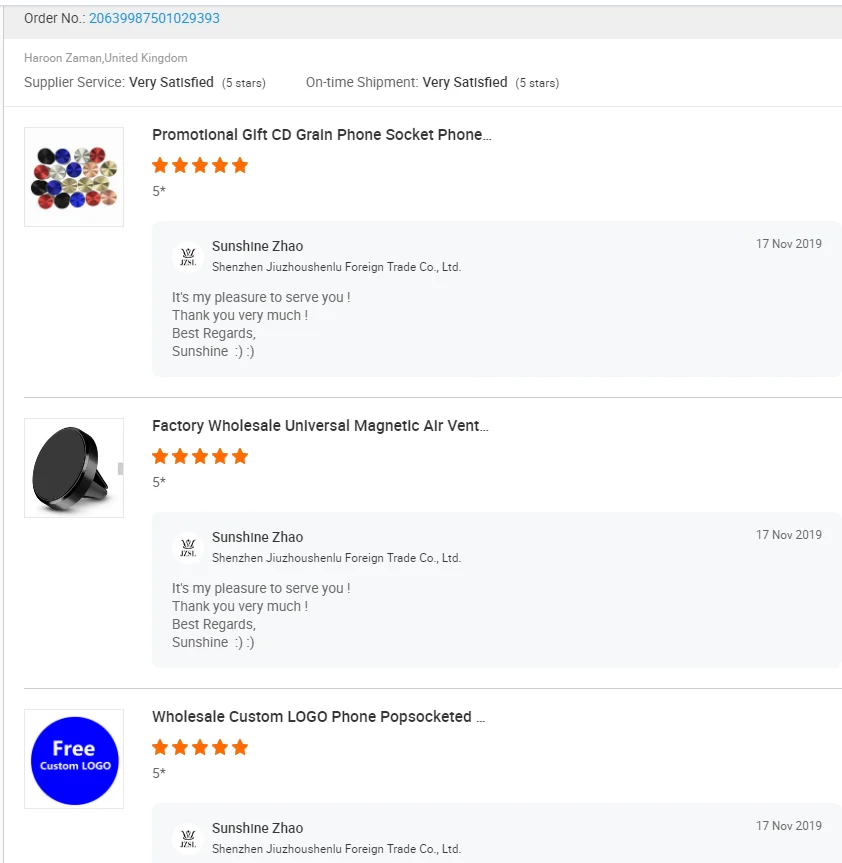The image depicts an order sheet, which appears to have been generated on a computer due to its organized layout and electronic format. At the top of the sheet, there is a prominent gray band displaying the text "Order Number," followed by the actual order number highlighted in light blue. The recipient's details are listed as "Haroon, Zayman, United Kingdom."

Underneath this header, the order sheet provides an evaluation of the supplier services, with Haroon rating both "Supplier Service" and "On-time Shipment" as "very satisfied," awarding five stars in each category.

The document is segmented into different sections. The first section is labeled “Promotional Gift” and includes items such as a CD, grain, a phone socket, and a phone. There is an illustrative square featuring round gems in various colors, presumably representing one of the promotional gifts.

Customer feedback is also featured, with a response from Sunshine Zhao, expressing gratitude and courtesy: "It's my pleasure to serve. Thank you very much. Best regards, Sunshine.” This section receives a five-star rating from Haroon.

Another section lists "Factory, Wholesale, Universal, Magnetic, Air Vent," which also mines a five-star rating with similar appreciative feedback: "It's my pleasure to serve you."

The final section, labeled "Wholesale, Custom Logo, Phone Pop Socket," also marks a five-star rating. This entry, however, has feedback that is cut off at the bottom of the document. This section features an image of the product described as a "Universal Magnet Air Vent," showing a black round device. Additionally, the custom logo is shown as a blue circle indicating "Free Custom Logo."

In summary, this detailed order sheet provides comprehensive information on the items ordered, their descriptions, customer satisfaction ratings, and appreciative messages from the supplier’s representative, Sunshine Zhao.